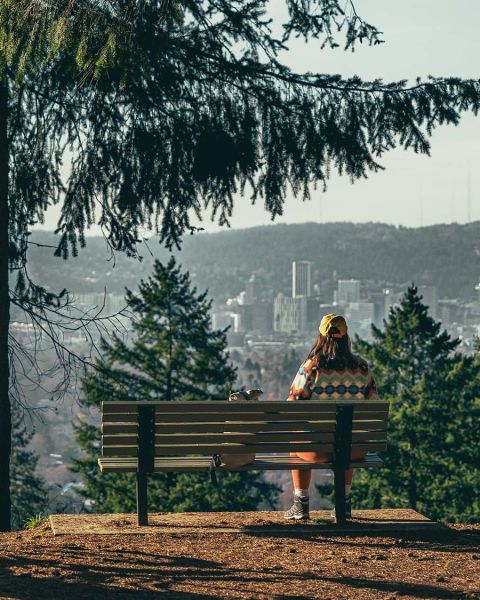This image captures a serene moment of a person sitting on a brown wooden park bench with black supports, positioned on a hillside surrounded by lush fir trees, likely in the Pacific Northwest. The individual, who has long hair and can be perceived as a woman, sits on the right edge of the bench, gazing over a cityscape nestled in a valley below. The person is dressed in a brown, green, and white sweater with matching pants, and gray tennis shoes. A yellow cap adorns her head, and an object, possibly a backpack, rests in the middle of the bench. The city, featuring predominantly gray and brown buildings, appears to be of moderate size, with its downtown area visible and a substantial hill providing a picturesque backdrop. The muted colors of the image, along with the shadows cast by the trees and the person, add a tranquil, almost introspective mood to the scene, enhanced by the hazy sky above. The overall composition places the viewer slightly behind and to the left of the person, sharing in her contemplative view of the harmonious blend of urban and natural landscapes.